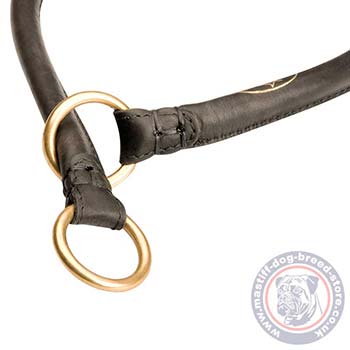This product image showcases a high-end, choker-style dog collar made of brown leather with a rounded cord design, intended to fit around a dog's neck. The collar features two gold-finished metal rings, adding a luxurious touch. The close-up view clearly shows the left side of the collar inserting through the metal ring on the right. This design allows the collar to tighten around the dog's neck when a leash, attached to the second ring, is pulled. The background is plain white, emphasizing the collar's details. In the lower right corner, there is a watermark featuring a circular image with light blue, red, and white colors, containing the face of a dog resembling a pug or St. Bernard. Encircling the dog image is a website URL: www.mastiff-dog-breed-store.co.uk.